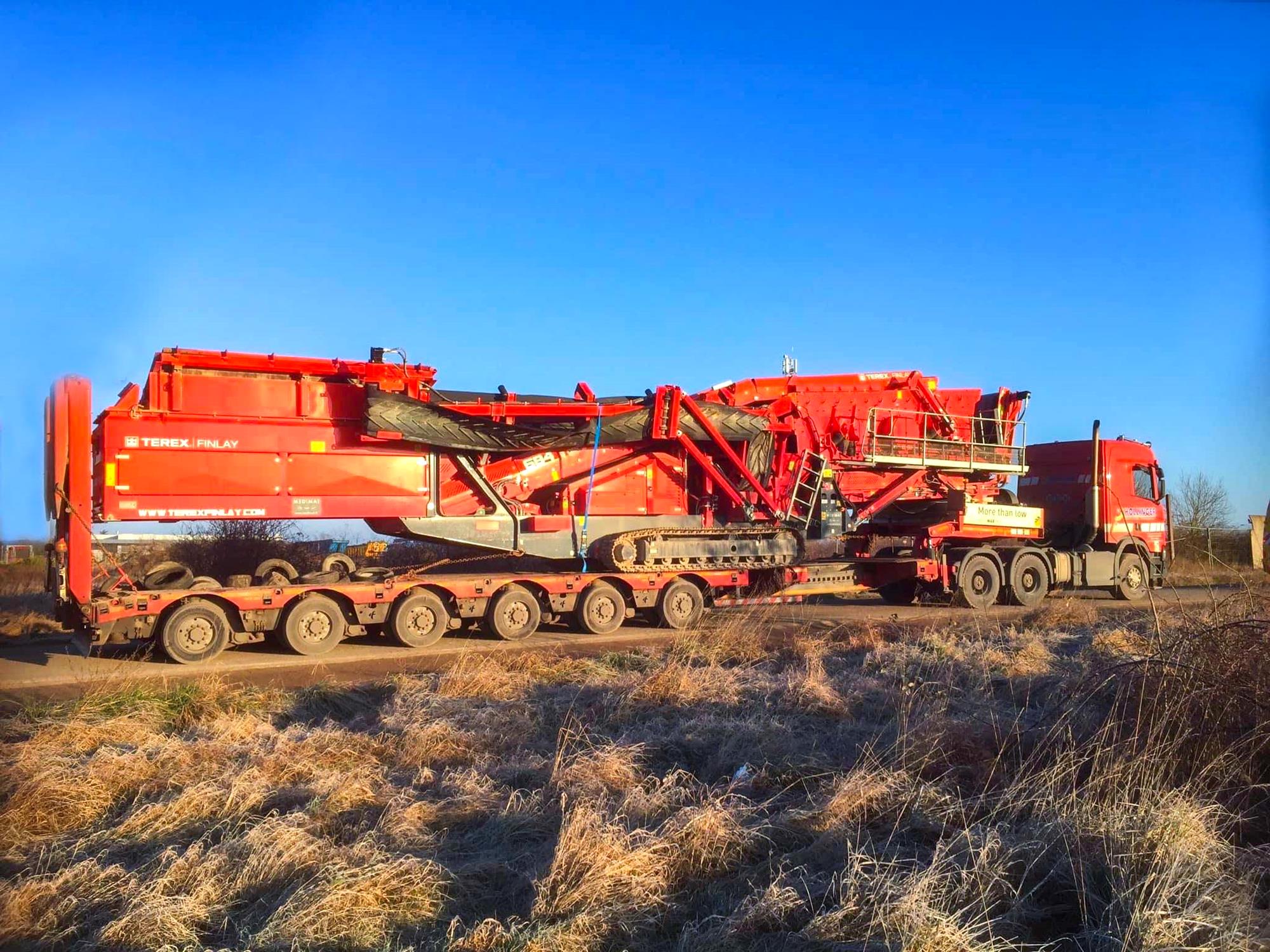The image depicts a bright daytime scene under beautiful, clear blue skies. A red, heavy-duty semi-truck with a very long, open bed is traveling on a flat, dark gray asphalt road. This semi-truck, a Tarex Finley, bears a large piece of machinery. The machinery, possibly an industrial processing or farm equipment, is painted red and has tank-like tracks at its base. It also features a conveyor belt on its side, guardrails, and an attached ladder, all in a metallic silver color. The road is flanked by dense patches of overgrown brown weeds and grass. The truck has a multitude of black wheels, with comments suggesting between 9 to 12 on each side, and carries spare tires on the back of the trailer. The equipment is securely strapped down with chains and tension cables, prepared for its oversized load journey.